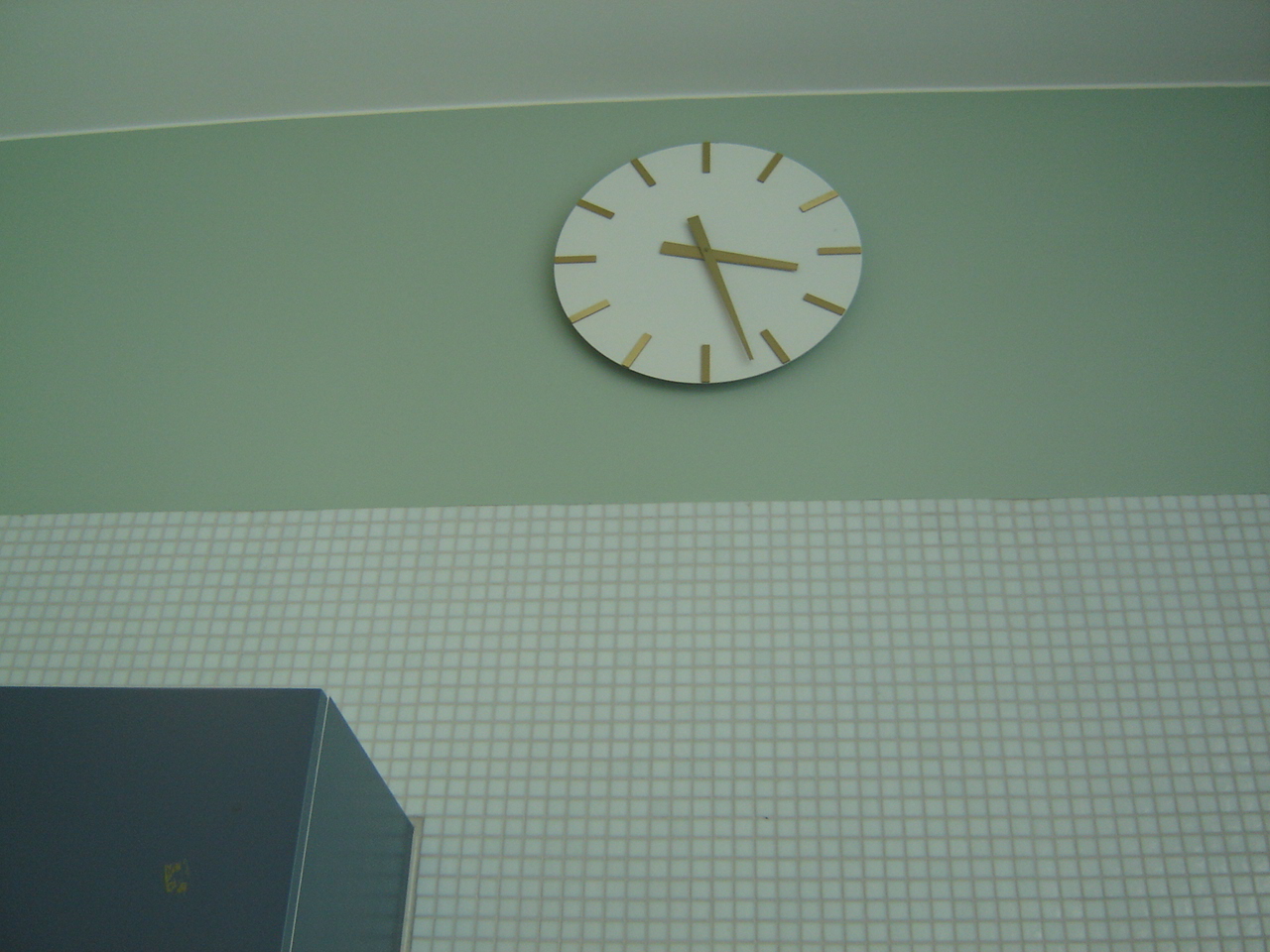In this evocative photo taken from a low angle, the viewer's gaze is directed upwards, capturing the intricate details of the wall and ceiling. The lower half of the wall is adorned with a grid of small, white squares separated by subtle, light-colored lines, suggesting a tiled or possibly wallpapered surface. Above this patterned section, the wall transitions into a smooth expanse painted in a soothing sage green. A crisp white line delineates where the wall meets the ceiling, which itself is painted a soft, light gray. Centrally positioned on the sage green wall is a striking white clock. The clock features elegant gold hands and minimalist gold lines in place of traditional numbers, adding a touch of sophistication to the decor.